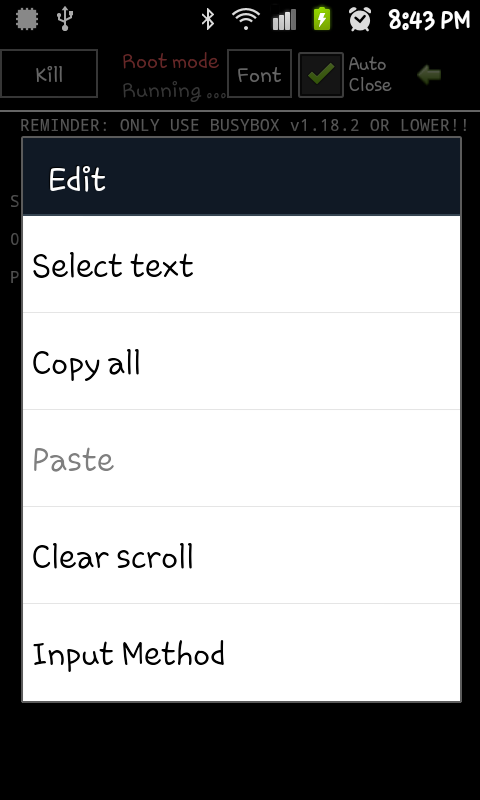The image depicts a screenshot taken from a cell phone, showcasing a software interface with multiple command options. The top of the screen displays various system icons, including signal strength, battery level, and notifications. Below this, there's a toolbar with several buttons and indicators. The uppermost toolbar features a "Kill" button, next to which is a notification in red text that says "Root mode" and "Running." Adjacent to this is a "Font" button followed by a green-checked square labeled "Auto Close." 

Beneath these elements is a reminder notice stating, "Only use busybox version 1.18.2 or lower."

The central section of the screen is predominantly white, contrasting against the black background, and takes up most of the display. This area provides several textual options: "Edit" (highlighted in blue), "Select text," "Copy all," "Paste" (grayed out), "Clear scroll," and "Input method." 

The font used throughout the interface resembles Comic Sans, which gives it an informal appearance, differing from the more polished and professional text usually seen in applications.